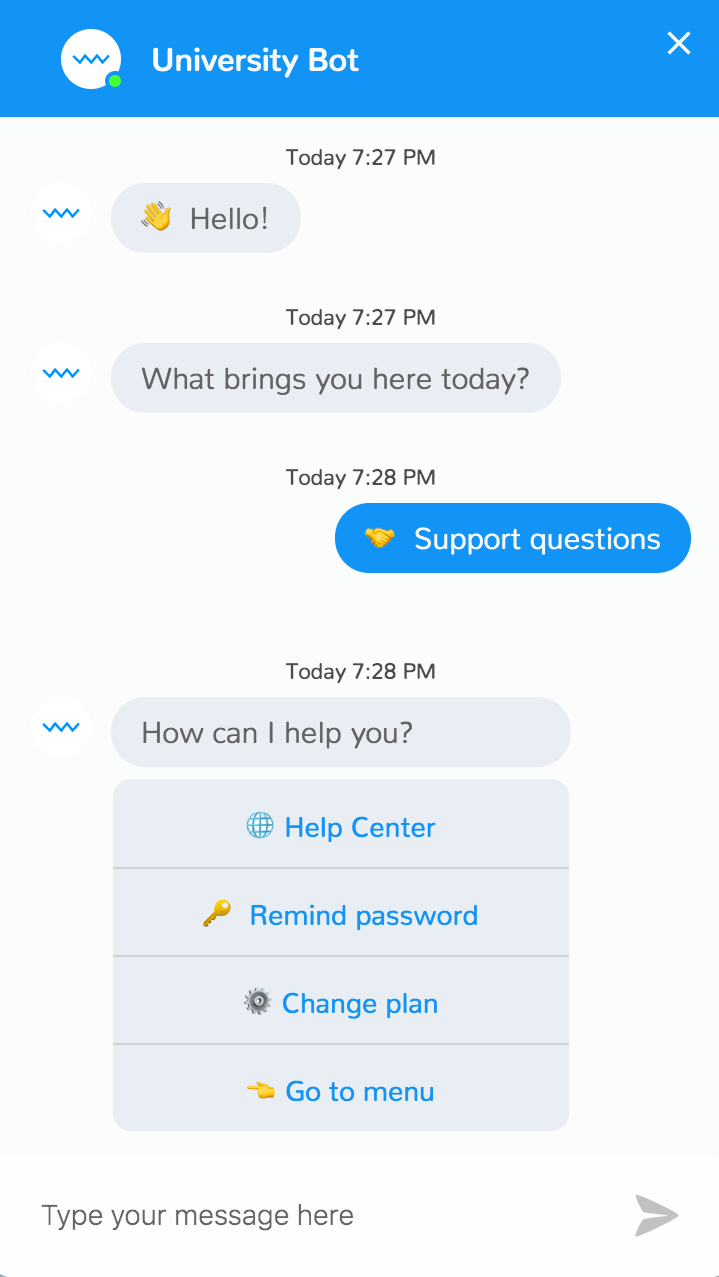**Caption:** 

The image depicts a simulated conversation with a chat bot, contained within a rectangular layout resembling a typical smartphone screen. The interface is predominantly monochromatic with shades of black, white, and medium blue. 

At the top of the screen, against a medium blue background, there's a header that reads "University Bot" in white text, slightly left of center. To the left of the text, there is a white circle containing a blue squiggly line resembling a series of connected 'W' shapes or waves. The bottom right corner of this circle has an aqua or teal green dot, and the upper right corner of the header includes a white 'X' for closing the chat.

Beneath this header, the main portion of the screen is dedicated to the chat conversation. The exchange starts with a timestamp in small, centered text at the top that reads, "Today, 7:27 PM." 

The first message from the chat bot, identified by the squiggly blue line on the left, appears in a light gray, rounded rectangle and reads, "Hello!" accompanied by a waving emoji.

The next bot message follows the same format, timestamped at "Today, 7:27 PM," asking, "What brings you here today?"

The human response, timestamped "Today, 7:28 PM," is right-justified in a medium blue, rounded rectangle with a handshake icon on the left, reading, "Support questions."

The bot responds again at "Today, 7:28 PM," in a similar format with the squiggly blue line on the left, saying, "How can I help you?"

Below this, a larger rectangular field with rounded corners presents four selectable options, each center-justified with an icon on the left. The options are: 
1. "Help Center" with a blue grid globe icon
2. "Remind Password" with a gold key icon
3. "Change Plan" with a gray and black gear icon
4. "Go to Menu" with a yellow hand pointing left

At the very bottom, a text input field is marked by the placeholder text, "Type your message here," shown in light gray in the lower left corner. On the far right of this field, there is a gray arrowhead pointing to the right, suggesting the capability to send a message.